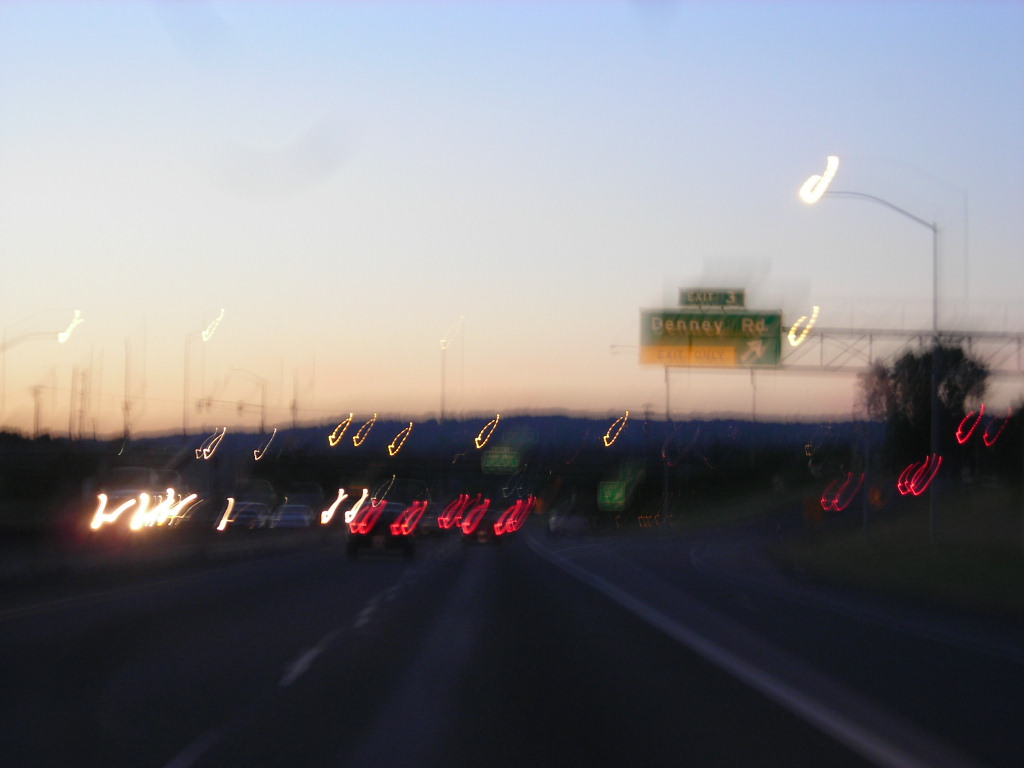A blurry image captures a highway scene from the driver’s perspective through the windshield, although none of the car’s interior is visible. The focus is on two lanes ahead, both flowing in the same direction. On the left side of the frame, lanes of oncoming traffic can be seen separated by a barrier. The photograph appears to have been taken during the twilight hours, with the sky showing hints of darkness as the sun sets low on the horizon, casting a subtle glow. A green exit sign is visible to the right, labeled "Exit 3" with "Denny Road" indicated above, and a smaller yellow section reading "Exit Only" accompanied by an arrow directing drivers to the off-ramp.